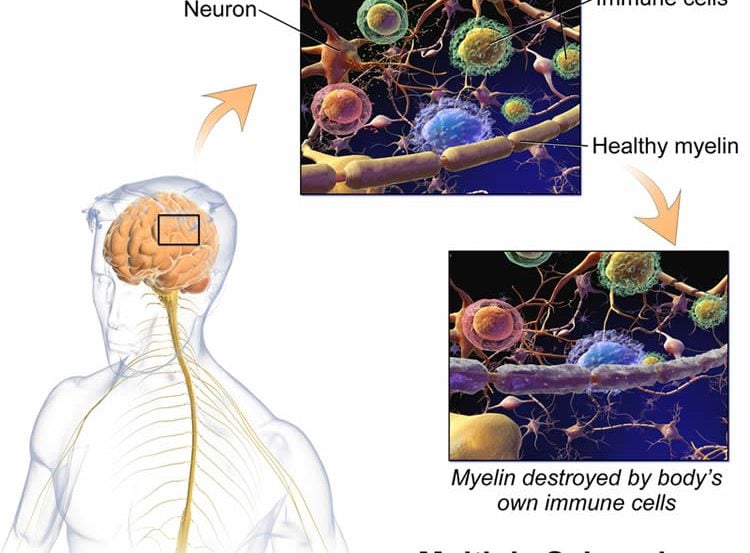In this detailed, scientifically illustrative image set against a white background, three images are arranged in a triangular formation to depict the human central nervous system and its pathology. On the lower left, a transparent, mannequin-like figure faces left, showcasing an inner view of the brain and spinal cord. This portion highlights the central nervous system with a square overlay pinpointing a specific brain area. An orange arrow extends from this square to the top image, labeled "neurons," with healthy myelin sheaths shown in yellow and neurons in orange. This top image features intricate details of neuron structures in various colors—yellow, red, blue, and green. However, a part of the image's label at the top is cropped out. The neuron image is connected by another orange arrow pointing downward to the lower right image, which depicts the detrimental effects of immune cells on the myelin sheaths, labeled "myelin destroyed by body's own immune cells." This comprehensive depiction is reminiscent of an excerpt from a scientific textbook, clearly illustrating the zoomed-in view of brain pathology and the impact on neural health through vibrant, informative diagrams.